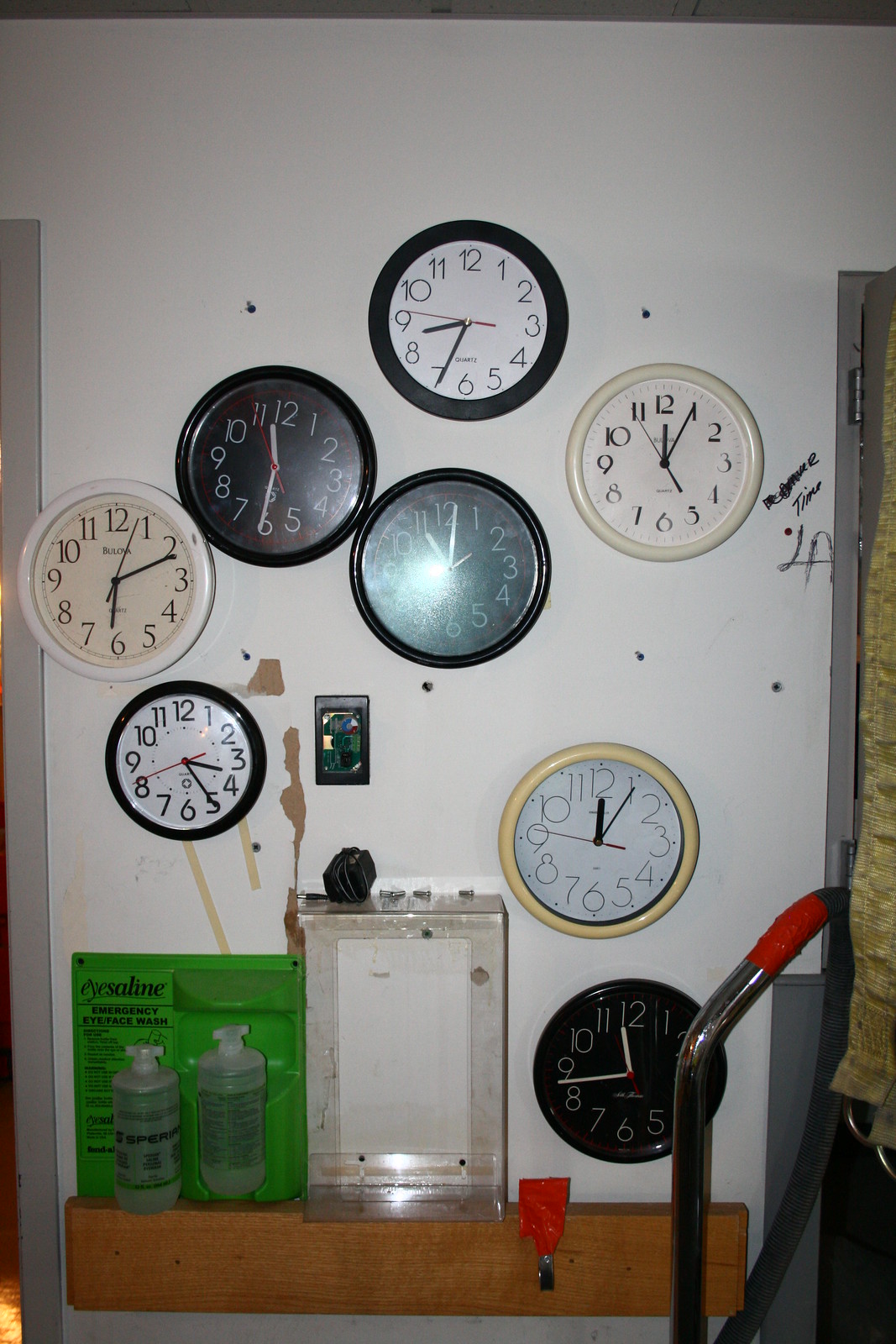This photograph displays a collection of nine diverse clocks mounted on a white wall, each clock distinct in its design and color scheme. The clocks are arranged in rows, showcasing variations in face color, numbering, and housing. Two clocks feature black faces with white hands and numerals. Another set of two displays white faces with black hands and a black outline. There are also two clocks with white faces bordered by white housings, with black hands and numbers. One clock stands out with a white face, beige outline, and black hands, while another has a taupe face surrounded by a rustic wooden housing.

Below the clocks, a light brown wooden shelf holds an assortment of items: two green-labeled plastic bottles containing a clear, slightly opaque liquid; a dark green bag with black writing that reads "iSaline" and "Emergency iBackside Space Wash"; and a white and silver square box. Adjacent to these, a metal handle with a silver finish and a red and black tip hangs beside the green-labeled bottles and a small metal box.

Altogether, this detailed image captures not just the multitude of clocks with their distinctive features, but also an array of uniquely placed items on the shelf, painting a vivid picture of the scene.